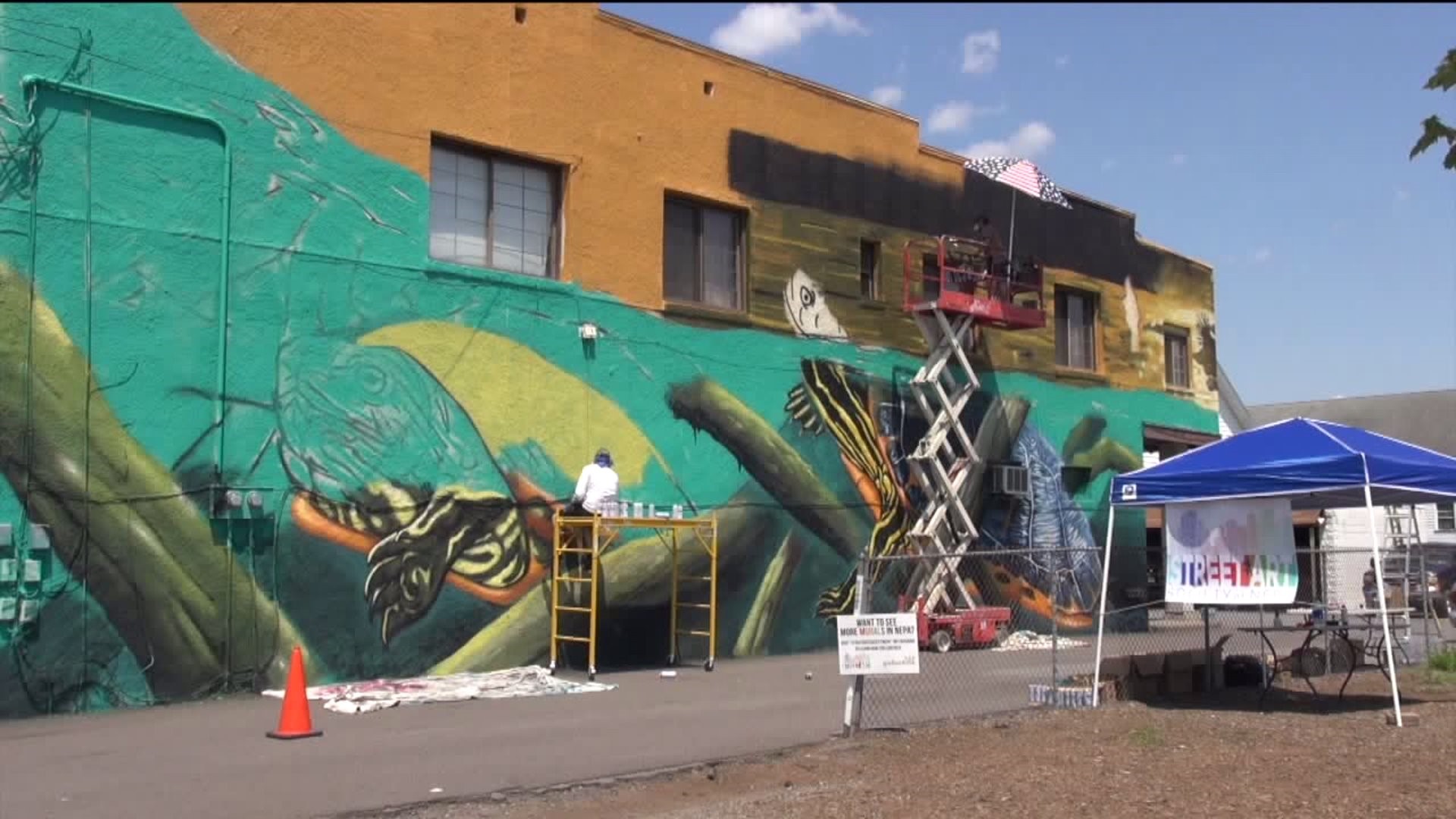A vibrant mural-in-progress of a serene ocean scene adorns the side of a large building in this photo. The mural prominently features a green-hued sea with intricate details, including a majestic tortoise gliding through the water and pieces of driftwood scattered naturally across the scene. Two men are hard at work on this artistic masterpiece; one artist is perched on a mobile lift, diligently painting the mural's finer details, while the other man is sketching additional elements. To the right side of the frame, a blue tent is set up, presumably housing supplies and providing a temporary workspace for the artists. The overall atmosphere is one of creativity and industriousness, capturing the mural's transformative journey from concept to completion.